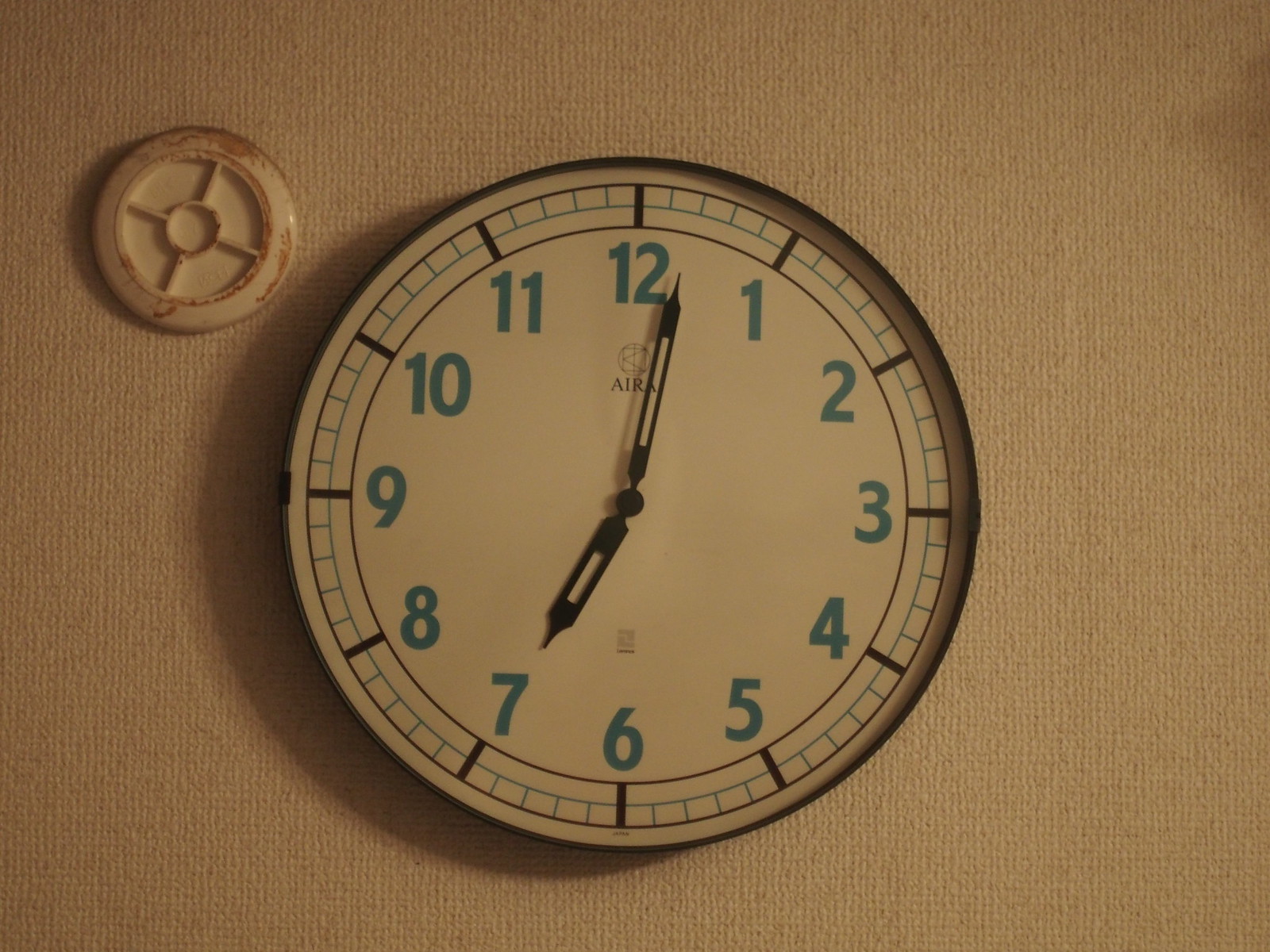The photo appears to be taken inside a residential setting, featuring an interior wall adorned with a light-colored fabric wallpaper that exhibits a subtle grid pattern. Dominating the center of the image is a large, round clock with a black outer rim. The clock's face is white, displaying bold blue numerals, and it has black hands indicating the time as 7:04. On the upper left-hand side of the picture, mounted on the wall, is a round plastic object of indeterminate function, adding an element of curiosity to the scene. The overall composition creates a sense of homeliness and subtle elegance through its choice of decor.